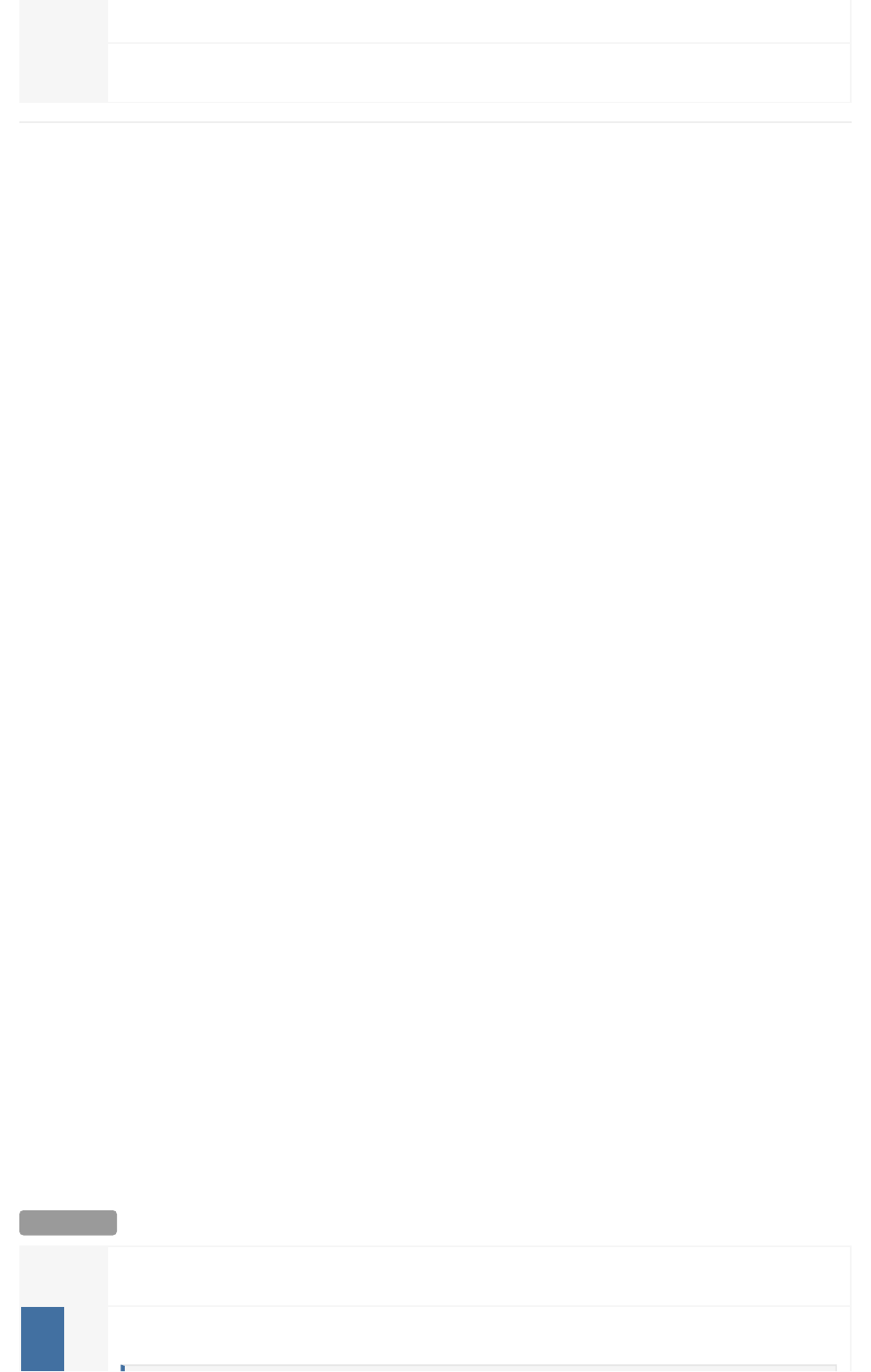In this image, we observe a predominantly white background with subtle details. There are no textual elements present. At the bottom of the image, a progress bar is visible, featuring a blue icon that indicates the current progress level, which suggests there is still a considerable amount left to be completed. The icons within the image are primarily rendered in grey and blue, standing out against the simplicity of the white backdrop.